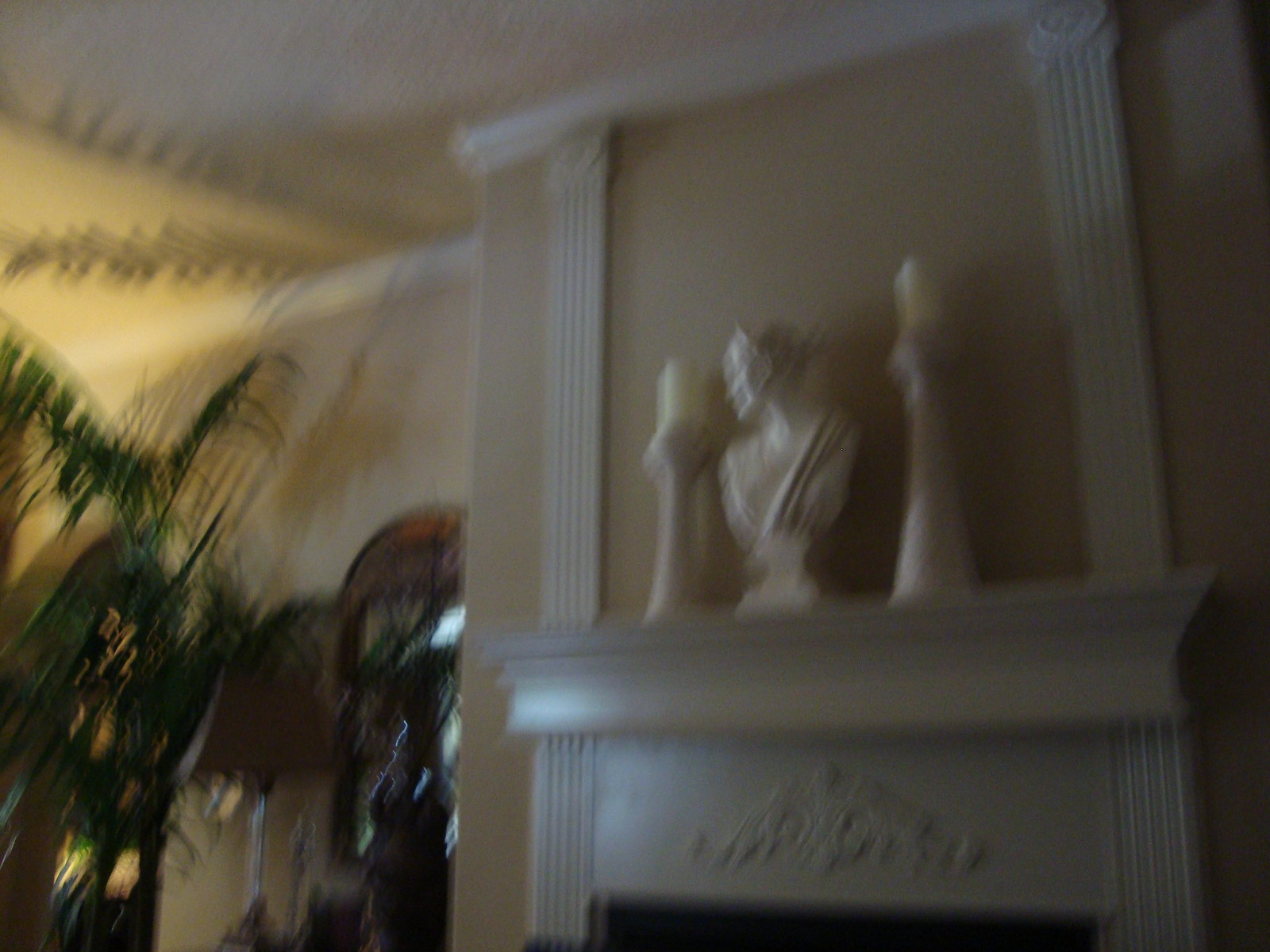Despite the blurriness of the photo, the setting of the image is discernible as an elegantly decorated room featuring a beautiful white fireplace. The mantel of the fireplace displays a striking arrangement: two tall, white candles, symmetrically placed, flank a white human sculpture that depicts a female figure with her hair pulled back, with the base of the sculpture artistically turned to the side. The wall behind the fireplace is painted in a soft, light yellow, providing a warm backdrop to the white decor. To the left of the fireplace, a leafy green plant brings a touch of nature indoors, while a lamp adds a layer of functionality and further decorative detail. The fireplace itself features a meticulously designed pattern on its back panel, enhancing the overall aesthetic appeal of the room.